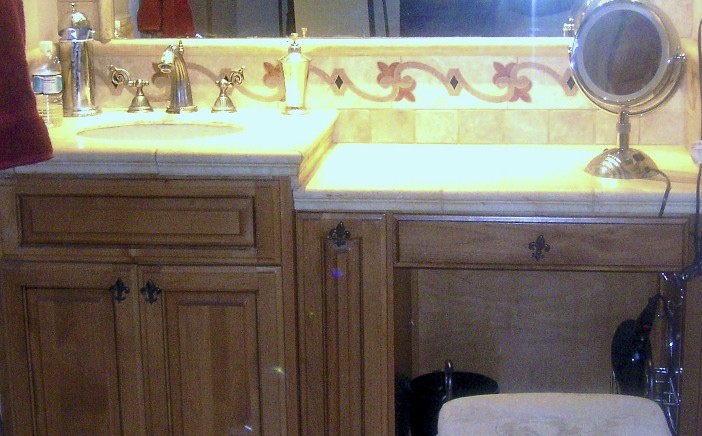This cozy and charming bathroom vignette features light brown cabinets adorned with sleek black handles. The cabinetry includes a central drawer and an open lower shelf that holds a white trash can. Various metallic and plastic items, along with a small black object topped with silver, hang from the open shelf. A pristine white countertop supports an oval-shaped sink with elegant gold fixtures.

A dual-sided mirror with a silver stand and a white-framed glass sits on the counter. The space is also accessorized with a red towel, a water bottle, and a couple of glass containers—one housing blue items possibly combs, and the other resembling a perfume bottle. Above the sink, a delicate backsplash showcases a light pink pattern with intricate ribbons forming diamond shapes accented with blue centers; the ribbons culminate in charming bow designs.

A large mirror positioned behind the counter reflects an assortment of clothing items and hints at a shower curtain in the background, completing the bathroom’s cozy and well-organized aesthetic.